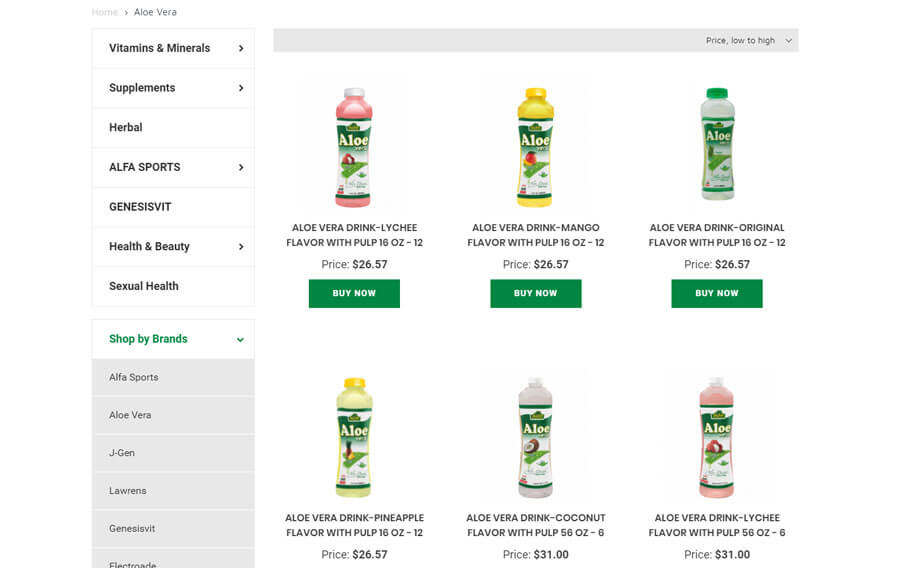The image showcases a detailed categorization of health and wellness products available in a store or online platform. At the top of the list are headings such as "Home," followed by "Aloe Vera," "Vitamins and Minerals," "Supplements," "Herbal," "Alpha Sports," "Genesis V.I.T.," "Health and Beauty," "Sexual Health," and "Shop by Brands." Brands listed include "Greg," "Alpha Sports," "Aloe Vera," "Jane," "Jen," "Lorenz," and "Genesis."

The products displayed are mainly Aloe Vera drinks, available in various flavors and packaging sizes ranging from 6 ounces to 12 ounces. Detailed descriptions and prices are provided for each flavor:

1. **Lychee Flavor with Pulp**: Pricing from $26.70 to $31.00.
2. **Mango Flavor with Pulp**: Price $26.70.
3. **Original Flavor with Pulp**: Price $26.70.
4. **Brown (possibly unflavored or unique flavor) Flavor with Pulp**: Pricing from $26.70 to $31.00.
5. **Coconut Flavor with Pulp**: Price $31.00.

Each product listing includes options to view in rich tones or buy now. The store interface allows sorting options such as price from low to high. The pink packaging highlights the Lychee flavor Aloe Vera drink, emphasizing its price in green for easy identification. The "Buy Now" button encourages immediate purchase for convenience.